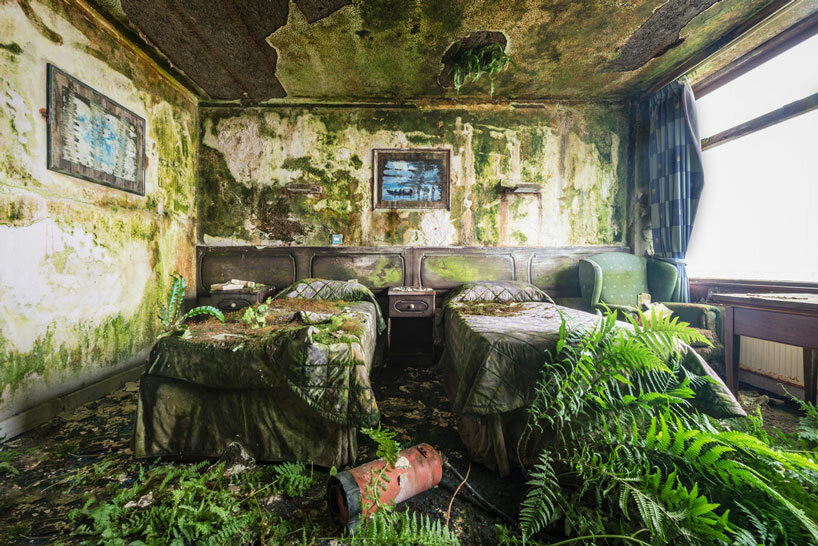The image depicts a dilapidated and abandoned bedroom with two beds that are heavily layered with dirt and various debris, surrounded by overgrown plants and ferns. The walls are a mix of white and green, now covered in dirt and moss. A red fire extinguisher is lying haphazardly between the two beds. There is a large window on the right, partially covered by an untouched blue and white checkered curtain, allowing light to spill into the room. Adjacent to the window stands a green chair, adding to the room's eerie ambiance. The ceiling is dirty and partially collapsed, with holes through which more vegetation can be seen emerging. A brown radiator is visible next to one of the beds, and there is a small table that remains surprisingly clean amidst the chaos. The overall scene suggests a sense of long-term neglect and natural reclamation, blending decay with resilient remnants of human habitation.